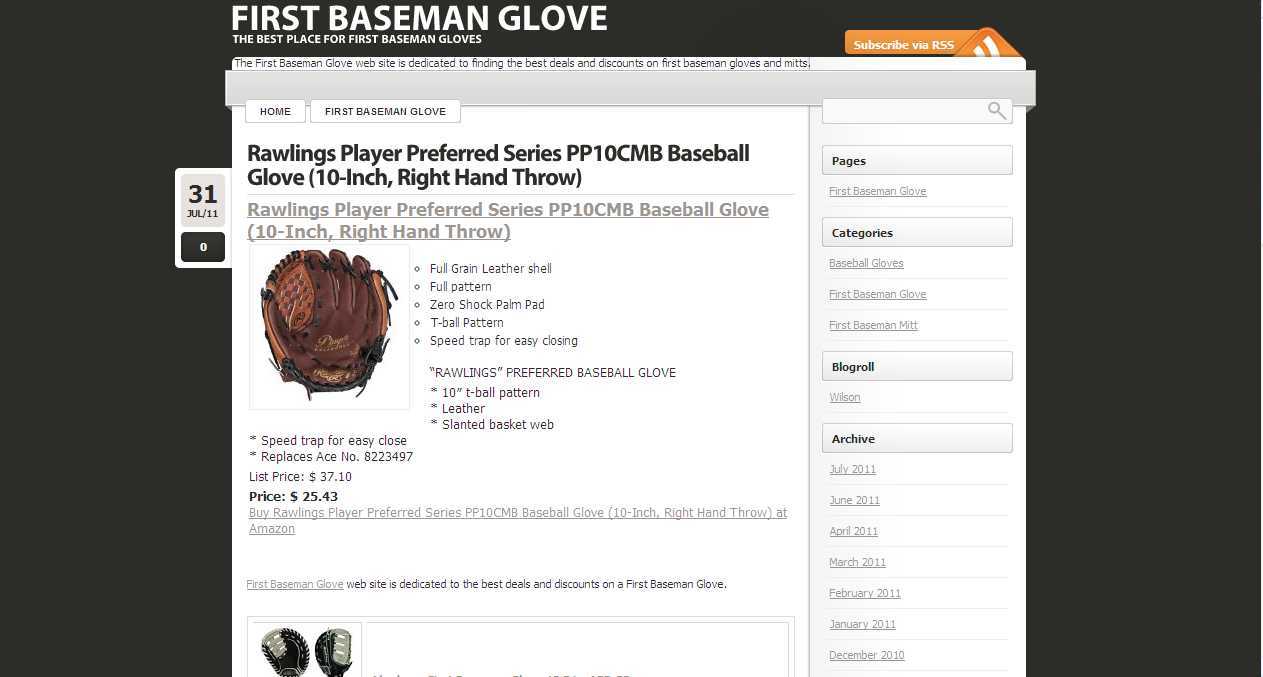The image depicts a webpage from "FirstBasemanGlove," a site specializing in first baseman gloves. At the top of the page, with a black background on either side, bold white text reads, "First Baseman Glove - The Best Place for First Baseman Gloves." The primary content is an information sheet showcasing a "Rawlings Player Preferred Series PP10CMB Baseball Glove, 10-inch Right-Hand Throw." This glove is made from full-grain leather, features a slanted basket web, a zero-shock palm pad, and a "Speed Trap" design for easy closing, ideal for T-ball. The glove, brown with black trim, is prominently pictured. Below this, additional details about the glove's specifications are listed in black text on a white background. Price details are also included, noting a discounted price of $25.43 from an original $37.10. The information sheet has an orange tab with white writing at the top and a smaller black-and-white tab on the side, marked "31." The layout also includes two small images of a black and gray glove at the bottom and navigation tags on the right side of the screen.